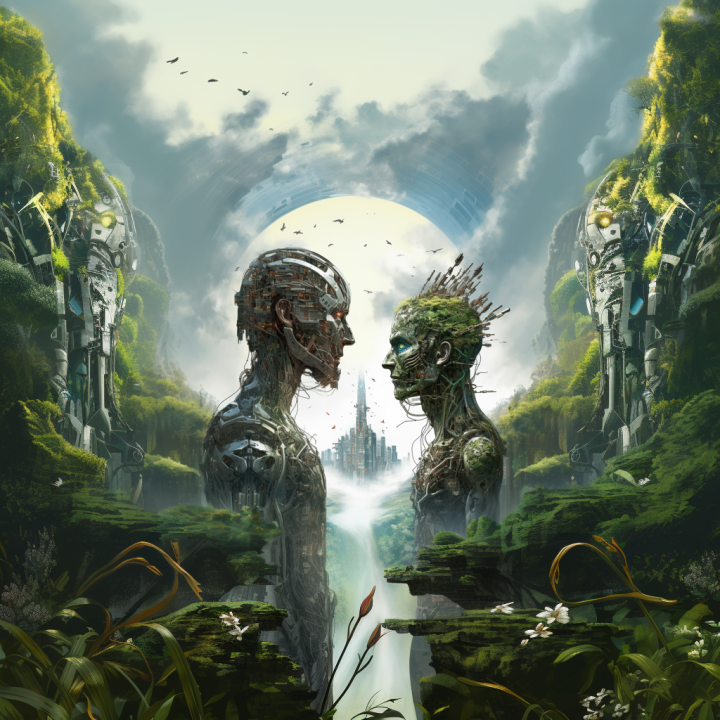This stylized, modern-looking painting depicts two intricately detailed robots standing face-to-face in the center against a backdrop that blends nature and technology. The robot on the right, slightly taller and appearing male, gazes downward at the female robot, who looks up at him. Both robots resemble androids with their outer skin removed, revealing an array of metal parts and wiring. The female robot features an interesting detail: a patch of green grass with tiny sticks protruding from it, resembling hair. 

Behind the male robot is a green mountain that slopes up and out toward the left corner, adorned with metal pieces emerging from its center. Similarly, a near-identical mountain lies behind the female robot, covered in green moss and trees with metal elements breaking through its core. The sky between the mountains is a gradient of blue and dark gray clouds, encircling the robots’ heads and extending down to their shoulders with a radiant halo effect. In the distance, there appears to be a futuristic city, or perhaps a castle, shrouded in mist. Additional details in the foreground include moss-covered rocks, white flowers, and pink flower buds, creating a canyon-like setting with walls composed of a mixture of foliage-covered rock and mechanical components reminiscent of the robots’ design.

The scene evokes the feel of a science fiction novel cover, merging organic and mechanical elements to create a compelling, otherworldly atmosphere.